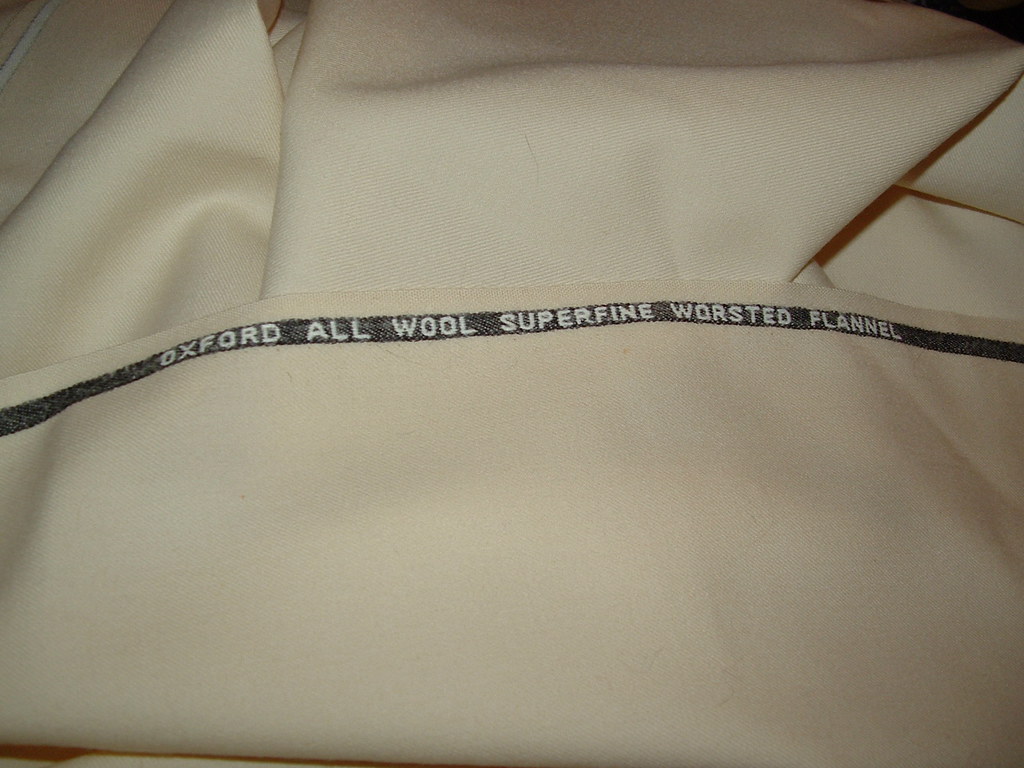The image features a large piece of cream-colored woolen fabric that appears to be a blanket or possibly a sheet set. This superfine worsted flannel material, labeled "Oxford all wool superfine worsted flannel" on a black strip sewn across one edge, is neatly folded in an unconventional manner with portions pulled up and laid over itself, giving it a wrinkled appearance. The creamy fabric is clean and consistent in color, with no variations or patterns. It is displayed on what seems to be a surface resembling natural wood, and the composition is highlighted by artificial lighting, likely from a camera flash, casting dark shadows in the background. The folded fabric suggests significant length, as it appears to be folded multiple times on both the sides and down the front.